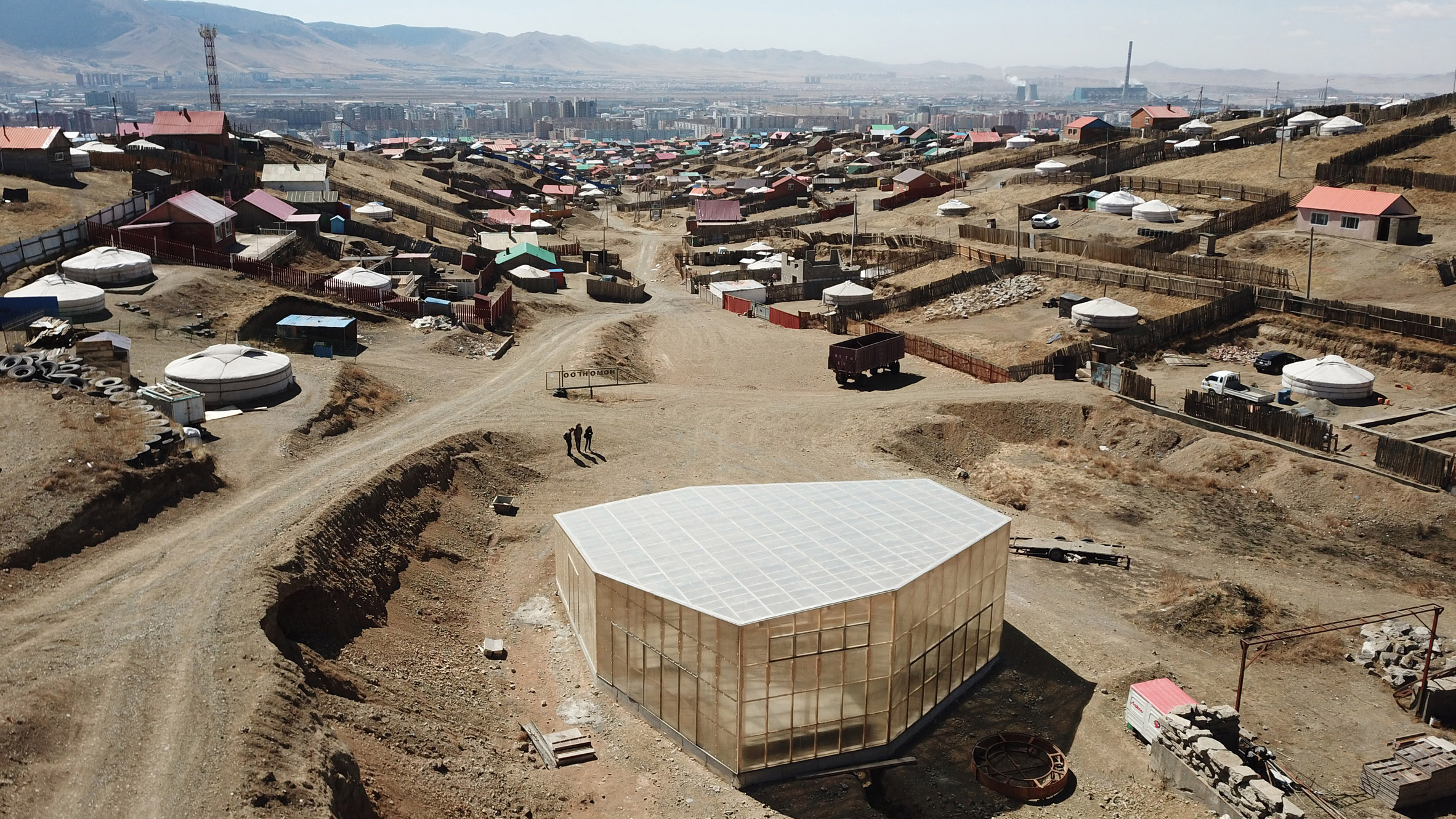The aerial photograph, possibly taken by a drone or low-flying aircraft, captures a desolate, sandy landscape that forms the backdrop of what appears to be a small village. The village is characterized by numerous round huts with pointed roofs, resembling small shelters, scattered across the area. Each hut is encircled by rudimentary fences made of posts, likely fashioned from tree limbs.

At the center of the image stands a unique glass structure with a polygonal, likely octagonal, shape featuring a solar-paneled roof. Three men are standing in front of this building, seemingly guarding it. The terrain is dominated by the brown, dusty ground typical of a desert-like environment.

Further in the distance, taller buildings rise on the horizon, suggesting the presence of a more developed area beyond this impoverished settlement. The sky above transitions from white to blue, and below it, a mountain range can be faintly seen in the far background, emphasizing the remote and arid nature of this locale. Scattered vehicles augment the depiction of a sparsely populated but inhabited village, possibly situated in a war-torn or economically challenged region.